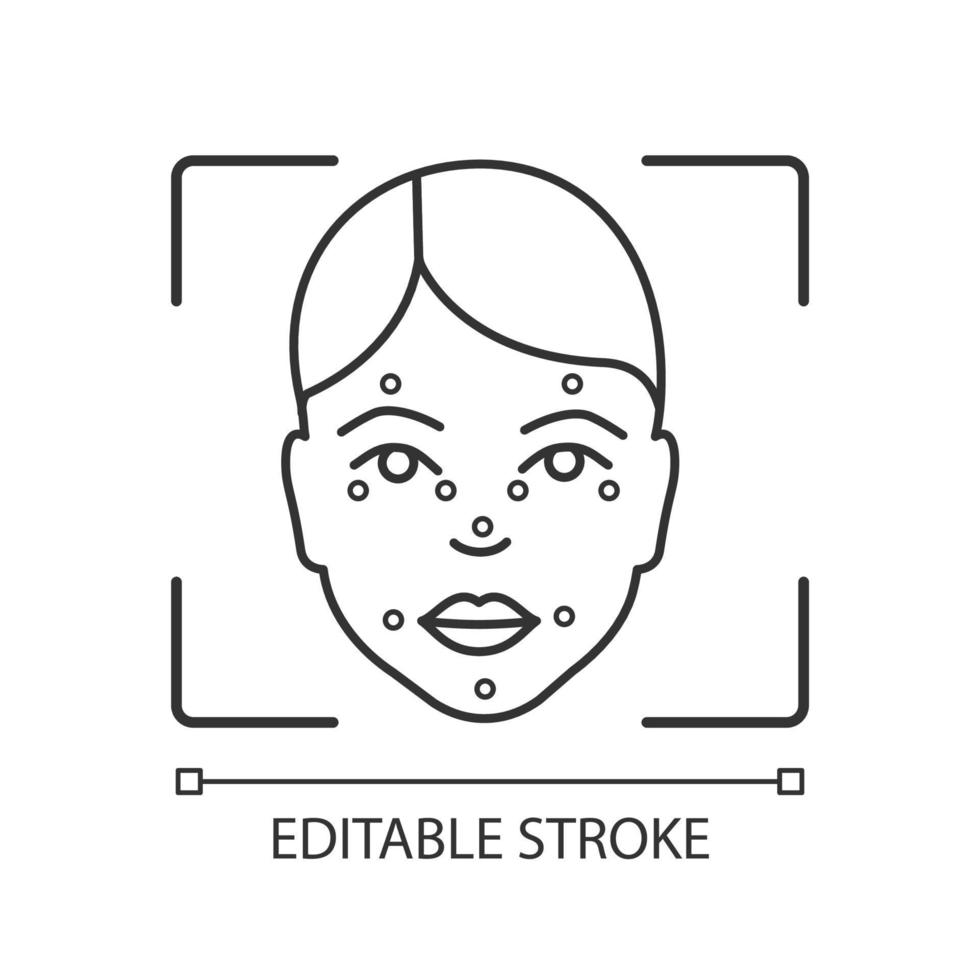This is a minimalist black and white drawing of a person's face, characterized by a simple yet expressive sketch. The face features thin, pressed-together lips, a small line for a nose, and clearly defined eyes and eyebrows. The hair is parted on the side, and where the ears would be, additional lines are visible. The face is adorned with several white dots with black outlines and white centers: one above each eye, one at the center of each eye, one on the tip of the nose, two on either side of the mouth, one on the chin, and two on the outer edges of each eye. 

The figure is framed within an irregularly shaped square with rounded corners, emphasizing the corners by filling them in with black. Below the face, there is a line flanked by two small square shapes, and the words "Editable Stroke" are written in all capital letters with a sans serif font. Despite its simplicity, the image is rich in detail and uniquely stylized.